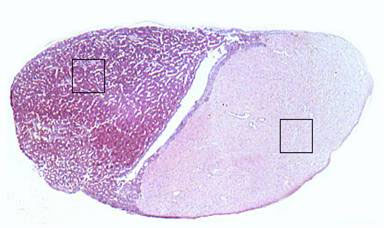This image showcases a cross-section of an oval-shaped object, reminiscent of a kidney bean or possibly a slice of ham, set on a white background. The shape is bisected by a vertical white stripe. On the left side, the color transitions to a dark pink or purple shade with fine white lines and features a small, black, square X in the upper portion. The right side of the shape is a lighter pink, again interspersed with tiny white lines. A small, black square appears towards the bottom right-hand side, seemingly focusing on a specific area within the light pink segment. The overall texture and appearance suggest a detailed, possibly medical image, capturing the intricacies of muscle or a similarly structured material, with distinct areas of interest marked by the black squares.